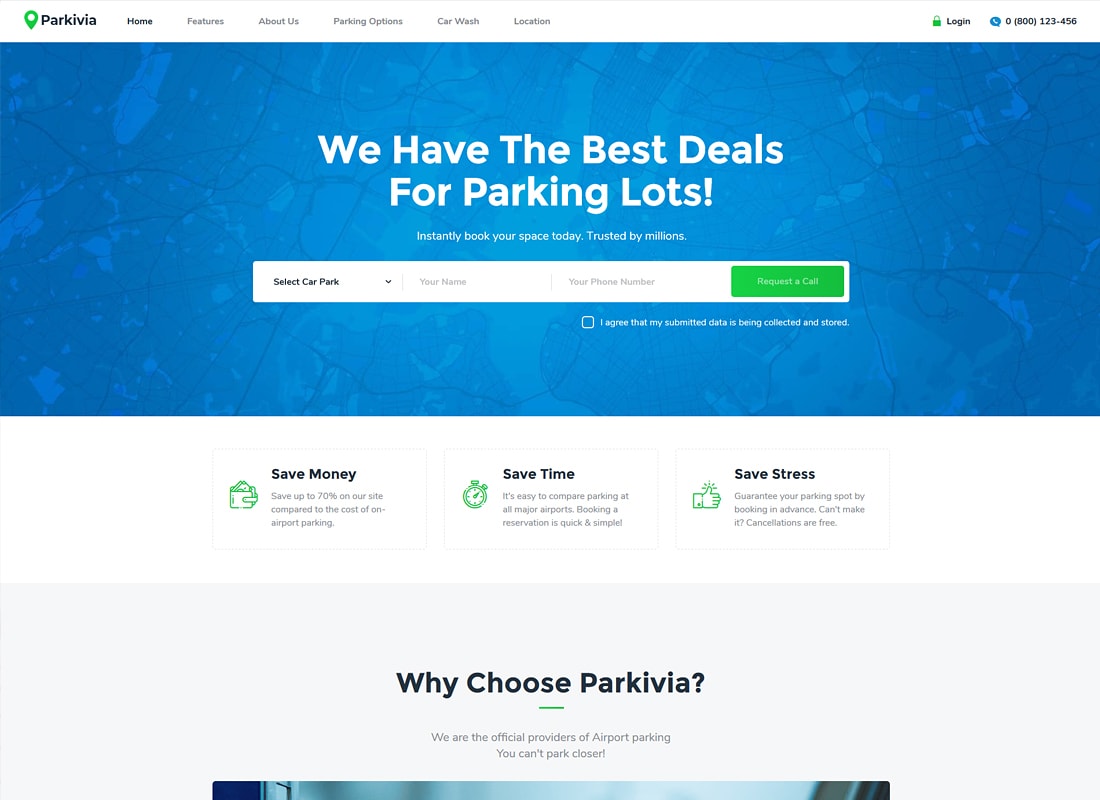Screenshot of the Parkivia Website:

At the top of the screen, the website's header features the logo "Parkivia" on the far left, followed by the navigation menu items: "Home," "Features," "About Us," "Parking Options," "Car Wash," and "Location." On the far right of the header, there are options for "Log In" and what appears to be a phone number.

Dominating the bulk of the screen is a large blue rectangular banner with the text: "We have the best deals for parking lots. Instantly book your space today, trusted by millions." Beneath this banner is a search bar prompting users to "Select Car Park," followed by fields for your name and phone number, and a button labeled "Request a Call." Small print indicates consent with, "I agree that my submitted data is being collected and stored."

Below the banner are three informational images, each with a distinct benefit highlighted:
1. "Save Money" - Save up to 70% on our site compared to the cost of on-airport parking.
2. "Save Time" - It's easy to compare parking at all major airports. Booking a reservation is quick and simple.
3. "Save Stress" - Guarantee your parking spot by booking in advance. Can't make it? Cancellations are free.

At the bottom of the screen, a section titled "Why Choose Parkivia?" declares, "We are the official providers of airport parking. You can't park closer."